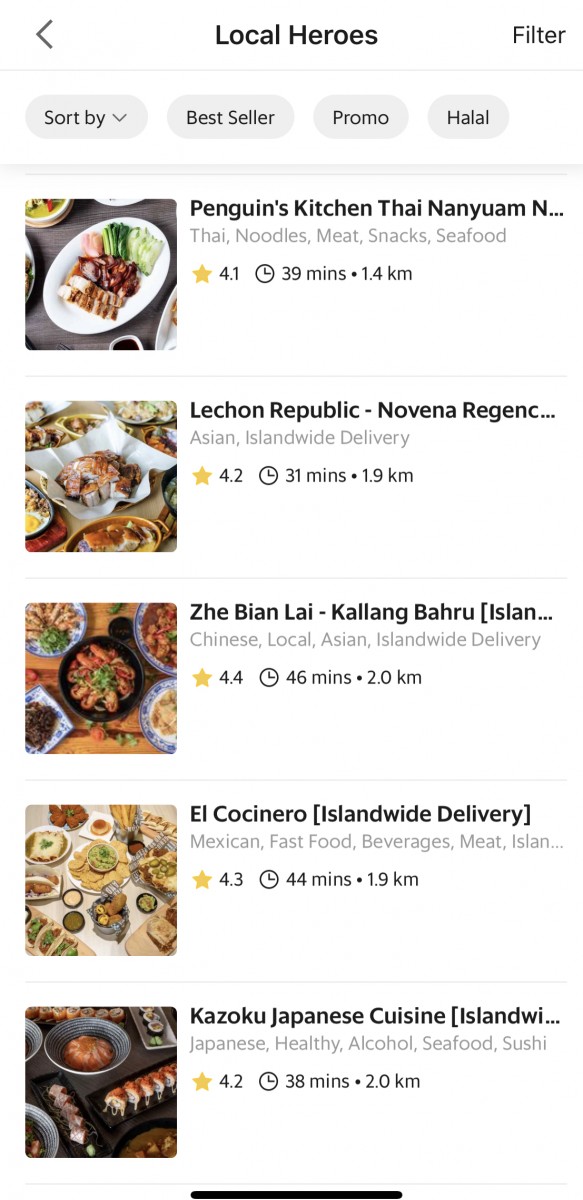The image depicts a screenshot from a food delivery app, which appears to be designed in a style similar to the Caviar app, recognized by its specific font and layout. Central to the interface is the "Local Heroes" section, showcasing local restaurants to help promote and support nearby businesses. This section includes a left arrow button for navigation and a filter option to sort through various choices. Below, a drop-down menu labeled "Sort By" is implemented, offering filters like "Best Seller," "Promo," and "How Loud."

The restaurant listings begin with "Penguin's Kitchen Thai Nam Yuen," featuring Thai cuisine such as noodles, meat, snacks, and seafood. This restaurant has a rating of 4.1, an estimated delivery time of 39 minutes, and is located 1.4 kilometers away. The accompanying image displays a plate of food with vegetables and what appears to be chicken.

Next on the list is "The Public Regency," an Asian restaurant with a 4.2 rating and a 31-minute estimated delivery time. The image here shows a possible assortment of sushi and bread.

Following that, a Chinese and local Asian restaurant offering island-wide delivery is listed, boasting a 4.4 rating and a 46-minute estimated delivery time. The image includes multiple dishes such as a vegetable roll dish, spring rolls, soup, and wontons arranged on a wooden table.

The fourth restaurant, "El Corserino," is a Mexican fast food outlet with a 4.3 rating and a 44-minute estimated delivery time. The image features a variety of items like chips with guacamole, tacos, enchiladas, and nachos, all scattered around.

The final restaurant showcased is "Fubuku," a Japanese cuisine restaurant. It has a rating of 4.2 and an estimated delivery time of 38 minutes. The photo includes sushi rolls, some type of bread in a bowl, and a soup dish.

Each restaurant listing includes a vivid image of their dishes, providing a visual taste of their offerings, encouraging the user to explore and support local culinary heroes.